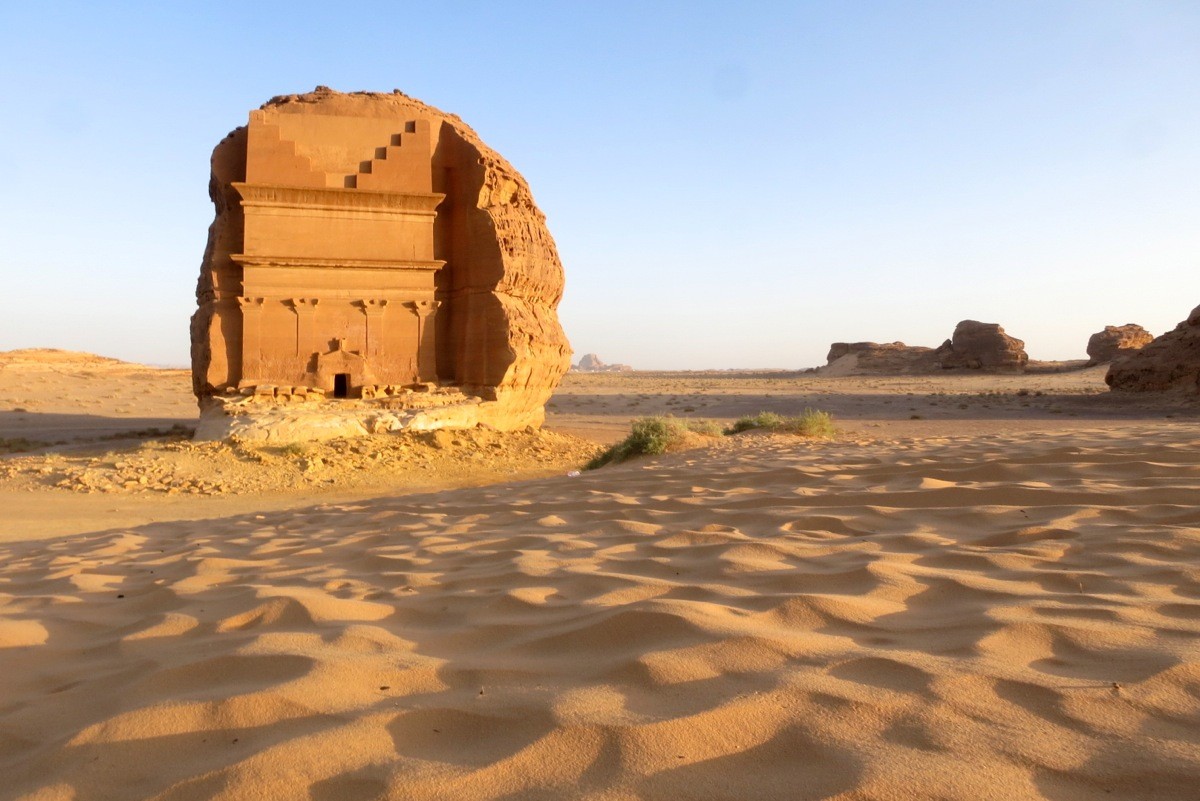This image captures an ancient ruin reminiscent of those found in the Sahara or Egyptian deserts. The scene is dominated by vast stretches of uneven, footprint-marked sand, punctuated by traces of green grass and small rocks. Central to the photograph is a partially destroyed stone structure, its intricate, sandy-colored walls appearing as if they were carved directly from the surrounding rock. This structure features a unique entrance at its base, invoking the impression of a building blending naturally into its rocky environment. Nearby, additional rock formations and ambiguous man-made structures enhance the historical aura of the site. The backdrop reveals a clear blue sky transitioning to white towards the right, adding to the serene, yet ancient atmosphere of the landscape.